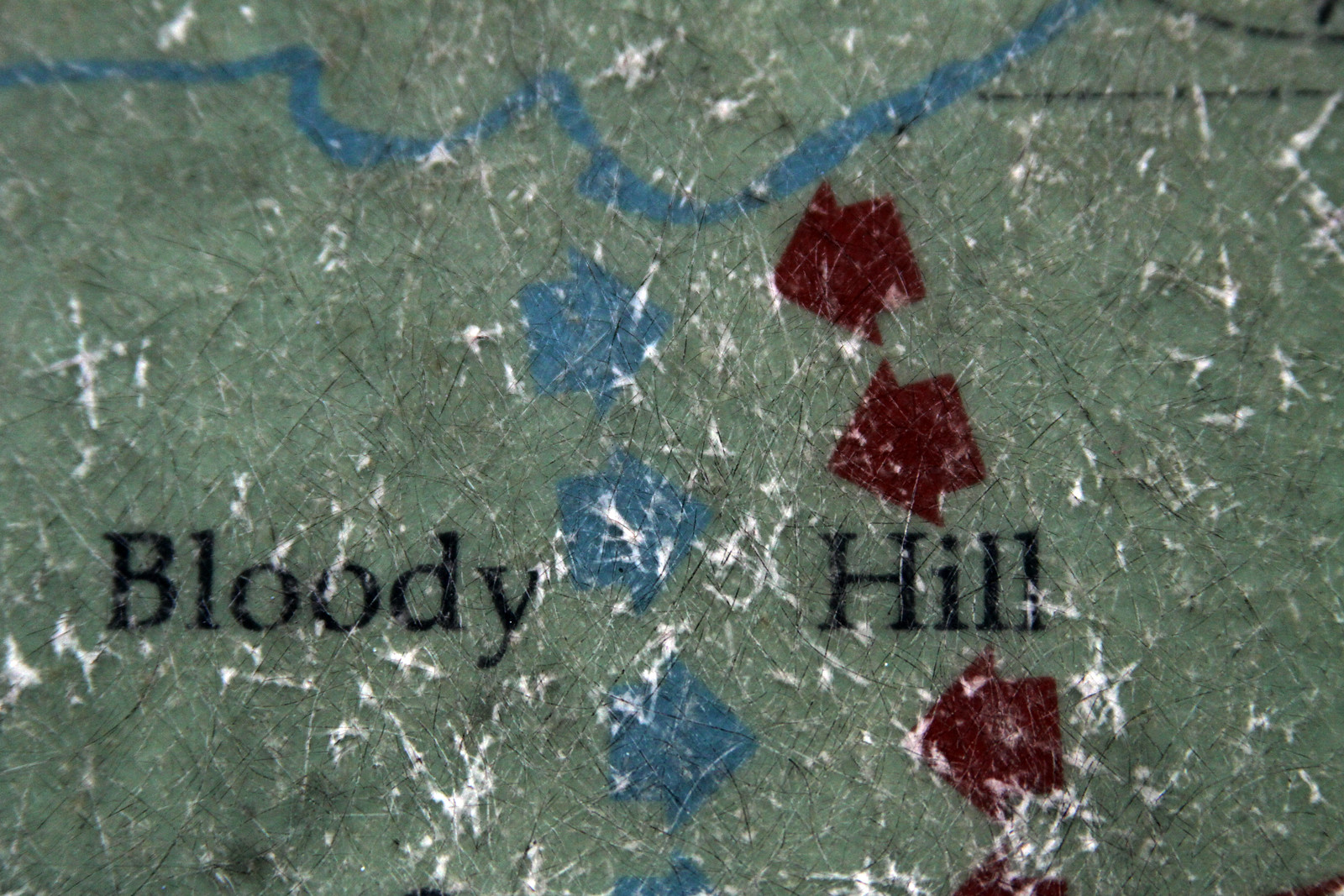The image is a rectangular, up-close view of a rough, worn-out map, likely depicting a military conflict. The main background color is a dull jade green, reminiscent of grass, with numerous scratches and pitted textures, giving it an aged, rocky appearance. Scattered white areas suggest paint chipping or wear. At the top, a blue streak meanders in a W shape, resembling a river, starting from the left corner and extending three-quarters across the top. Central to the map is the label "Bloody Hill" in black print. Below this, there are two sets of arrows: three blue arrows on the left side pointing right, with a fourth partially visible at the bottom, and four red arrows on the right side pointing left. The map appears to be made from a material like metal or plastic, indicated by its uneven, rough surface.